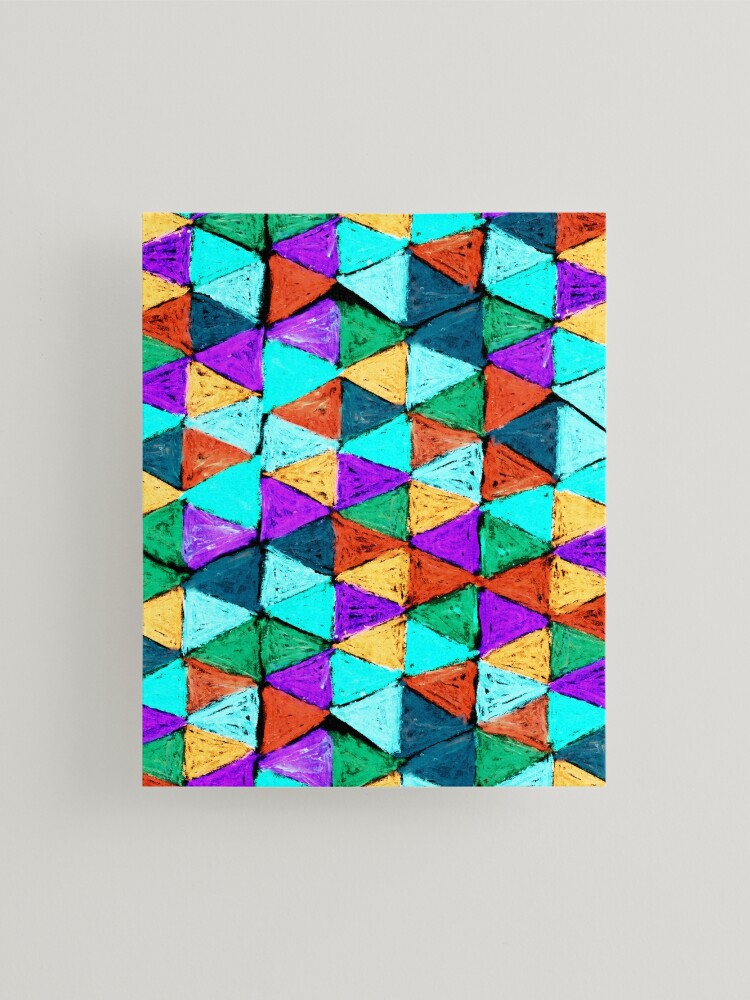The photograph depicts a vibrant piece of artwork displayed in an art gallery or museum, mounted on a plain gray wall. The artwork is rectangular and heavily features interconnected, multicolored triangles that span the entire canvas. The triangles exhibit a rugged, scratchy texture that suggests the medium might be oil pastel or chalky substance. Predominant colors include dark purple, yellow, red, green, dark blue, vibrant light blue, teal, ember orange, and burnt yellow. Brushstrokes are visible within the triangles, indicating it might also be an acrylic or oil painting. The visually striking array of triangles, organized in three main rows or columns, come together to form a diamond-like pattern that fills the entire space of the artwork.